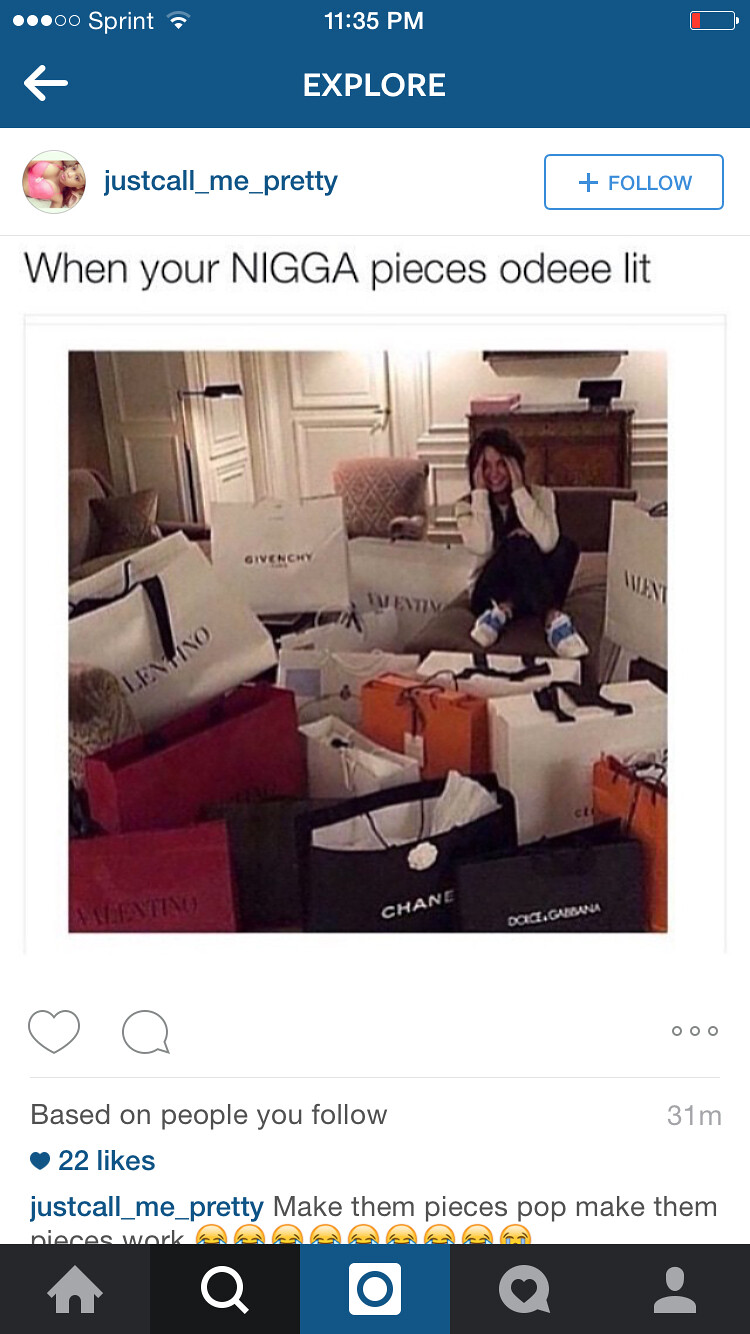The image is a screenshot from a cell phone, displaying a post on a social network. At the top of the screen, a blue band with white text reads "Explore," and adjacent displays indicate it is 11:35 PM, with the carrier being Sprint and battery life displayed. The upper left corner also shows a partial message notification.

The central content is a post by the user _just_call_me_pretty_ featuring a photograph of a young woman seated on the floor of a living room, surrounded by numerous luxury shopping bags from high-end brands such as Givenchy, Valentino, Chanel, and Dolce & Gabbana. The caption on the post, written in black text, states, "When your nigger pieces OD lit." The woman is holding her hands to her temples, suggesting an overwhelming or ecstatic emotion.

Below the image, some cut-off commentary is visible, indicating the post's popularity, with 22 likes noted. At the very bottom, a black bar shows the standard navigation buttons of the smartphone, including home and search icons.